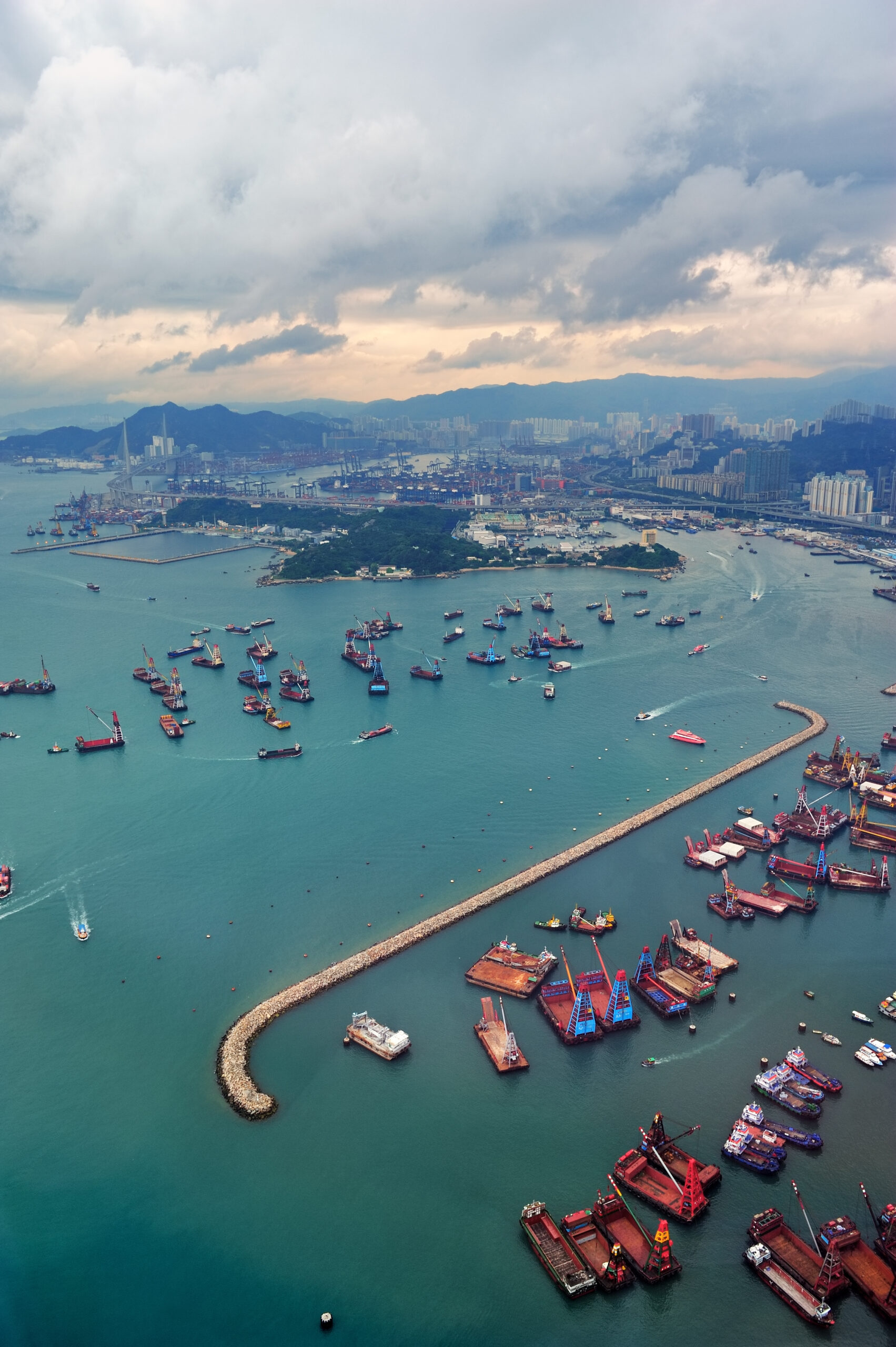The image captures an aerial view of a bustling marina nestled at the edge of a vibrant city. In the foreground, a variety of boats, including open-top ones in red and blue hues, float on bluish-green water, creating a lively scene. Towards the right, a long, hook-shaped dock stretches out, accommodating about ten vessels, and potentially serving as a sandbar or other structural feature. Farther out, the marina extends with more barges and ships navigating the water, leading the eye towards the midground's lush green island adorned with trees. The city's skyline, composed of small, possibly industrial buildings and taller structures, meets the water’s edge and is framed by a range of mountains to the left. The sky above is laden with clouds, suggesting a cloudy, possibly stormy ambiance that adds a dramatic backdrop to this picturesque harbor.